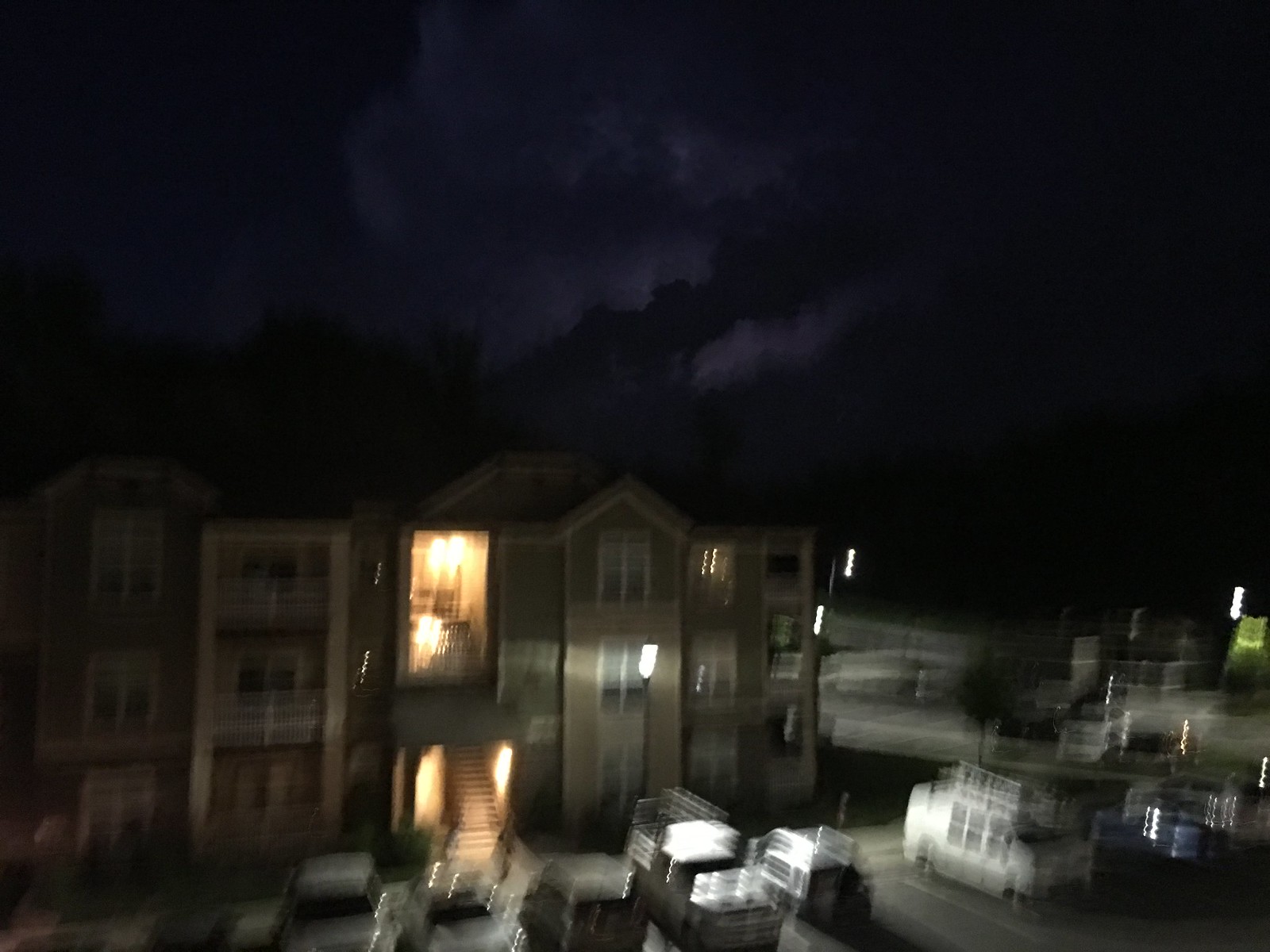A dark, blurry nighttime image captures the scene of a three-story hotel, possibly located in a rural area. The sky, a dark blue with a couple of hazy, lighter-blue clouds, sets a somber backdrop. In the distance, a mountain range with discernible tree shapes lines the horizon.

The hotel appears to be either tan or gray in color. Distinguishing features include a peaked roof above one window, resembling an upside-down V, alongside numerous flat roof sections. Central to the structure is an illuminated outdoor stairwell, open and devoid of doors, lit by bright yellow lights, indicating a common access point for reaching the upper floors.

To the left of this stairwell, the building features two balconies with white railings and sliding glass doors; similar structures are present on the right side and at least on the first floor. 

In a gray, indistinct parking lot in front of the building, seven vehicles are parked, including a large minivan and a truck, although the specifics are difficult to discern due to the image's overall blurriness.